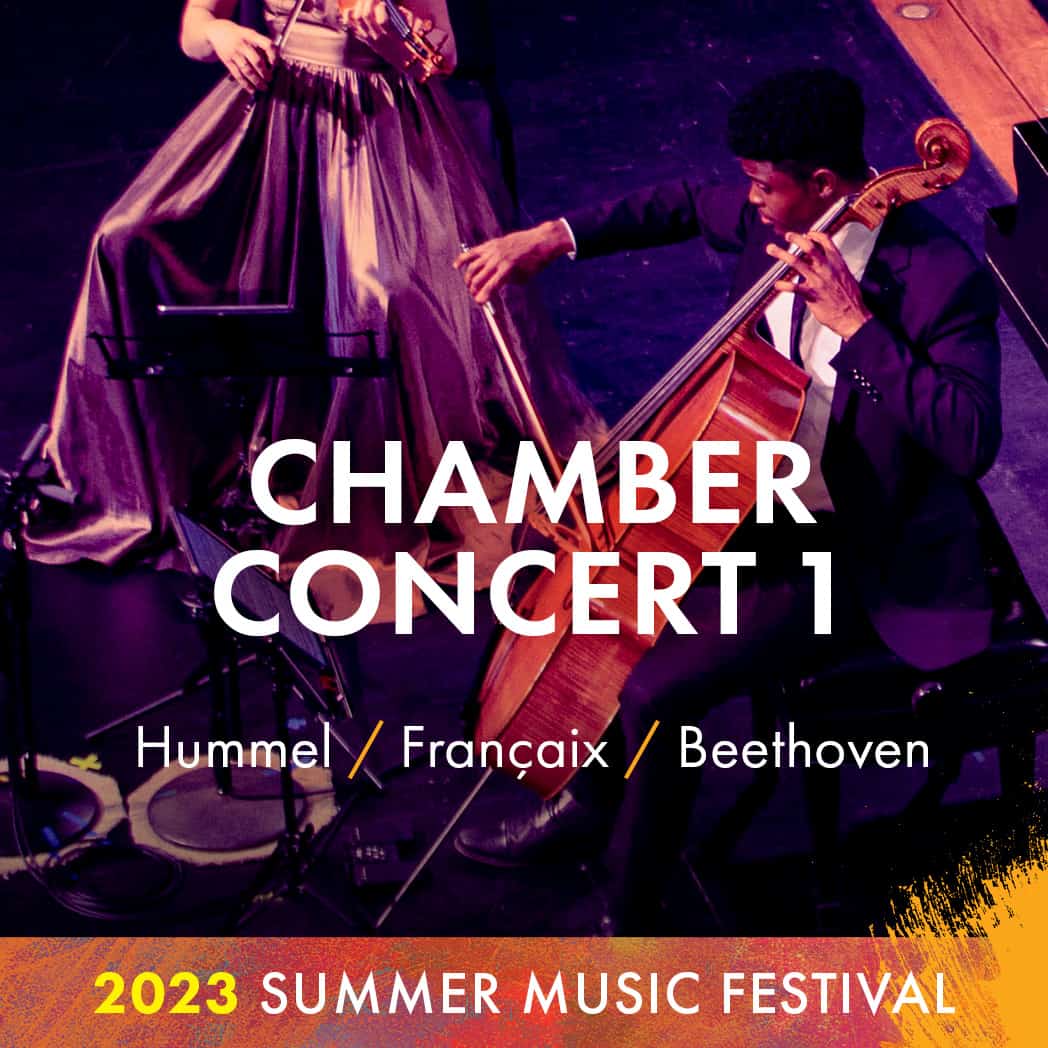This promotional image for "Chamber Concert No. 1" showcases an African-American man with a high top fade, dressed in a casual suit with a bow tie, playing a cello. The text "Chamber Concert No. 1" is centrally placed in white type, with the names of the featured composers—Hummel, François, and Beethoven—listed beneath it. At the bottom of the image, the caption reads "2023 Summer Music Festival." To the left of the cellist, there is the lower half of a woman seated, playing a violin, with her purple silk skirt flowing down. Her head and upper body are cropped out of the frame. The background features a dark ground with a wooden plank detail and subtle hues of blue and purple, adding a rich, vibrant tone to the composition.